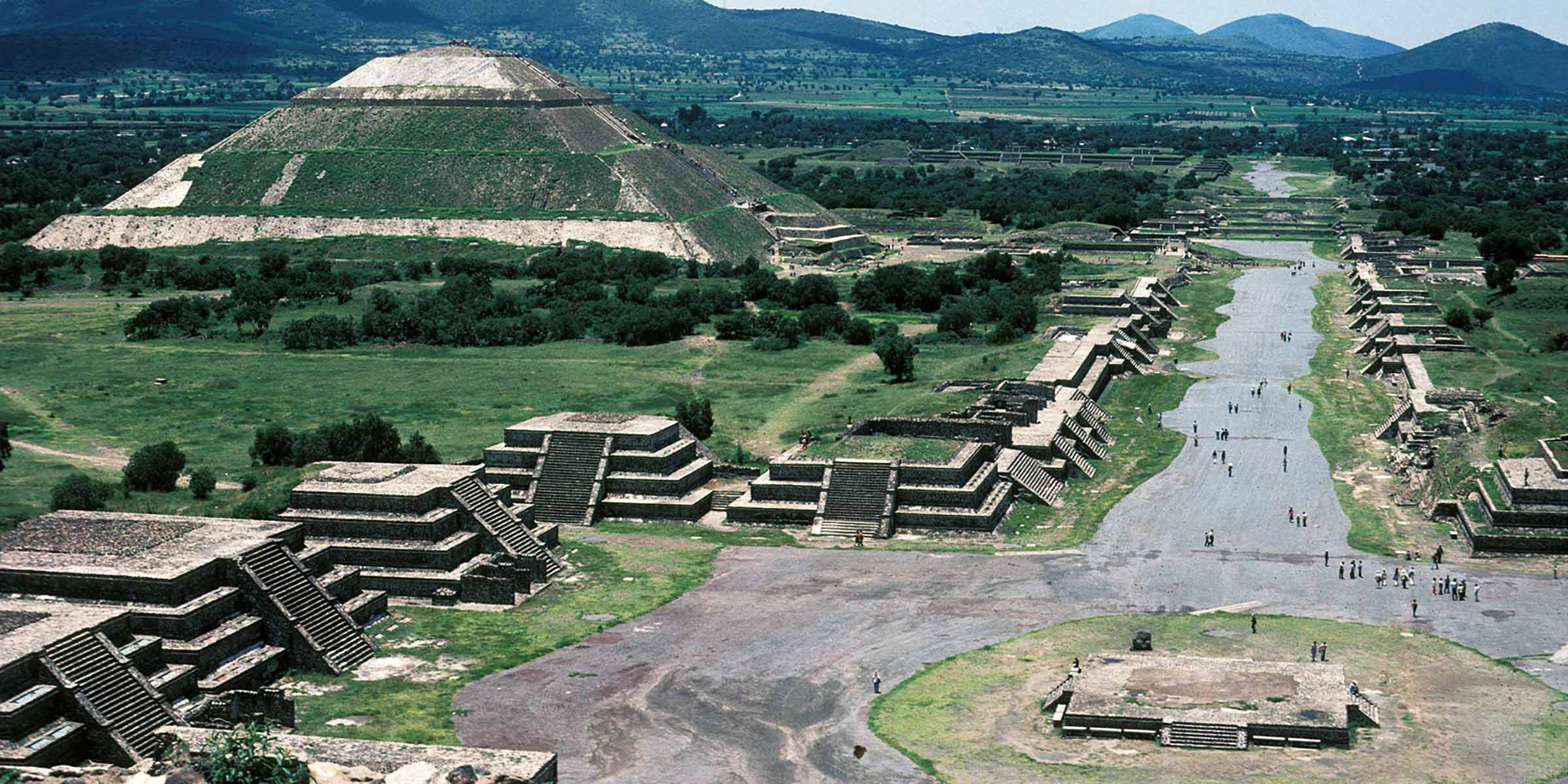The image depicts a vibrant, sunlit scene likely situated in central or southern Mexico, dominated by ancient Mesoamerican pyramids, likely ziggurats built by the Aztec civilization. The point of view is elevated, almost aerial, capturing a complex archaeological site. In the background, a sprawling mountain range is visible, wrapped in green foliage and juxtaposed against a partly visible blue sky in the top right.

Centrally, a massive pyramid with distinct, broad staircases commands the upper left section of the image, surrounded by several smaller pyramids arranged in a semi-circular layout. These pyramids feature multiple levels, with staircases leading up their sides. At the bottom left, four smaller pyramids align neatly in a row, with a fifth to the side. The bottom right of the image shows a circular area housing a small platform-style structure.

A weatherworn, uneven dirt or clay road runs through the site, looping around the central structures and connecting various points of interest. This road appears to gravel or stone in certain sections and is flanked by open spaces with patches of grass and clusters of green trees, which are particularly prominent on the left side of the image. Tourists meander along the road and explore the ruins, enhancing the image’s lively and historical atmosphere.